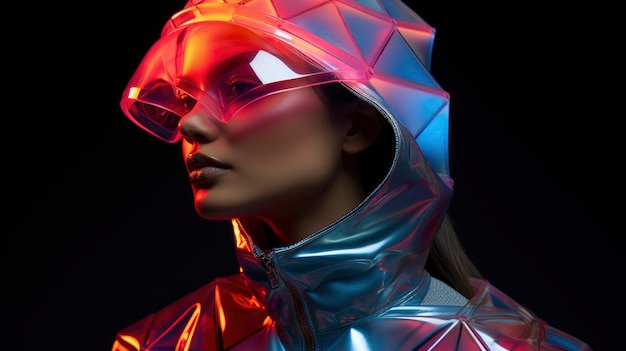The image is a realistically rendered, hyper-resolute piece of digital art set against a black background, depicting a dark-complexioned woman adorned in a futuristic metallic hoodie. The hoodie, constructed from interconnected triangular and trapezoidal shapes in various shades of metallic silver and blue, features pink neon highlights along the edges that fade into a vivid visor rendered in neon yellow, orange, and pink hues. This visor acts as a protective shield for the woman's eyes, while the lower part of her face, including her well-defined jawline, high cheekbones, and impeccable brown skin, remains unobstructed. She has traditional female features with glossy lips and what appears to be a ponytail emerging from the back of her suit. Her attire, which covers her from head to her upper shoulders, includes a zipper that extends to her lower throat. The left side of her body is illuminated by a pinkish-orange light, enhancing the neon accents of her suit and visor. The woman is posed looking to the left, occupying the center of the image from top to bottom.